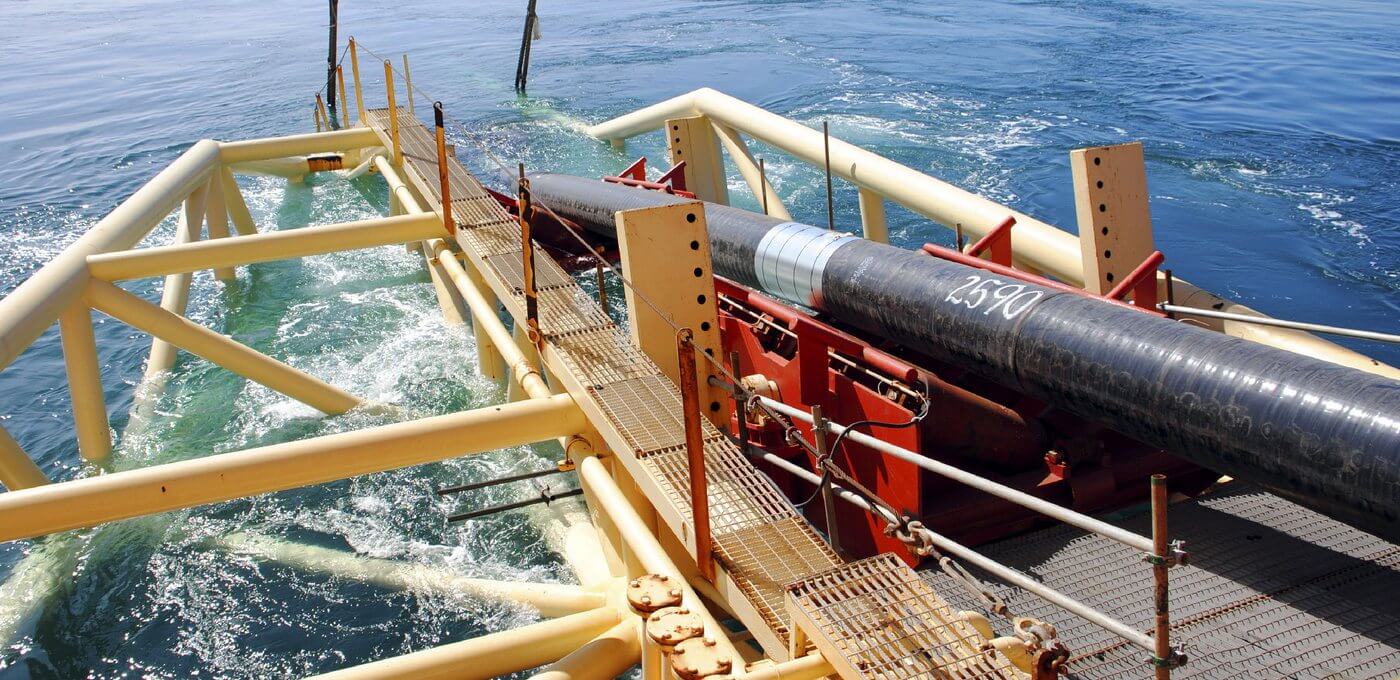In the photograph, we observe an oceanic scene featuring a beige-colored vessel equipped with a yellowish-ivory metal scaffolding, which includes walkways and railings. The water beneath is a vibrant blue, transitioning to green in some areas, with visible white foam indicating movement. Central to the image is a long, black metallic tube, resembling either a drainage pipe or a small submarine, marked with the numbers 2590. This tube is extending from the vessel into the water, appearing to either submerge or be constructed to channel something into the ocean. Supporting this structure is a red underpinning that bolsters the pipe, adding to the intricate metal framework. The overall impression is one of a complex maritime apparatus under a bright and sunny sky.